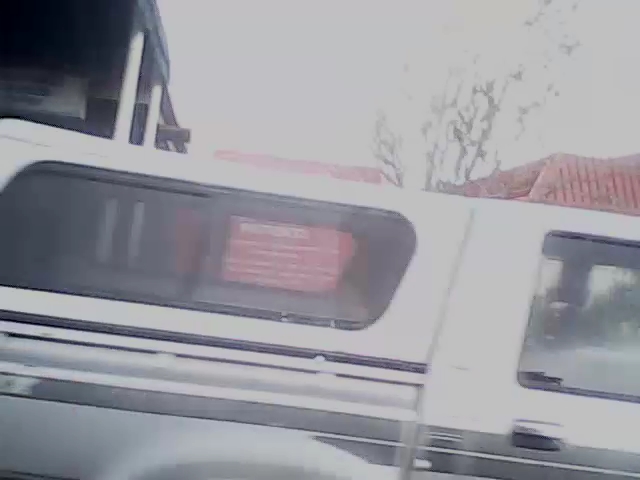The image depicts a white pickup truck with a large camper top occupying the rear. The truck features a prominent black stripe running horizontally along its side and rubber molding around the windows, extending from the front to the back of the camper top. The picture, which might have been taken in motion, provides a sense of movement from left to right in the outdoor setting. A light grey, blurry sky forms the background, along with multiple structures. One building has a flat red roof and a partially visible red sign, though the sign's text is unreadable. Another taller building, with blue trim and white support posts, rises behind the truck. This structure appears to have a classic tilted roof and might be casting a shadow over the scene. A spindly tree with noticeable leaves can also be seen in the distance. The overall scene is slightly blurry, suggesting it might have been captured from a moving vehicle.